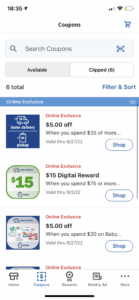This is a blurred screenshot, seemingly taken from a mobile phone, displaying a shopping or coupon app interface, likely Kroger. At the top, the time is shown as 18:35, with location services enabled, 2 bars of signal strength, full WiFi, and a low battery indicator. The main header reads "Coupons," featuring an option to search for available coupons and a count of 6 total clipped coupons. 

There are filter and sort options in blue. The list of coupons includes:

1. **Online Exclusive** - $5 off when you spend $35 or more.
2. **Online Exclusive** - $15 digital reward when you spend $75 or more.
3. **Online Exclusive** - $5 off when you spend $20 on baby products.
4. Another **Online Exclusive** coupon, but the details are cut off.

At the bottom navigation bar, icons indicating "Home," "Coupons," an unclear third option, "Weekly Ad," and a "More" option represented by an ellipsis are visible. Additionally, a small blue shopping cart icon is present next to the "Coupons" header.